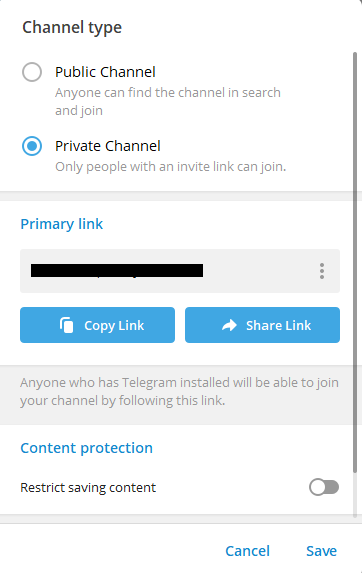This screenshot appears to be from a messaging or social media application, likely Telegram, depicting settings for creating or managing a channel. The interface is divided into several sections. At the very top, there are options labeled "Channel Type," with descriptions for "Public Channel" and "Private Channel." The "Public Channel" option notes that anyone can find and join the channel via search, while the "Private Channel" option, which is currently selected, restricts access to those with an invite link.

Beneath this, there is a section for the "Primary Link," which has been blacked out for privacy reasons. Following this, there is functionality to "Copy Link" and "Share Link" allowing users to distribute the invite link, ensuring only those with Telegram installed will have the ability to join the channel.

Further down, there is an option for "Content Protection" where users can "restrict saving content." However, the slider button indicating this feature is currently in the off position and not selected.

The bottom part of the screenshot shows "Cancel" and "Save" buttons, presumably for the user to either discard or save their settings changes.

There are no visual or photographic elements in this image, nor does it contain any human figures, animals, plants, vehicles, or buildings. The focus solely remains on the text and interface elements of the settings menu.